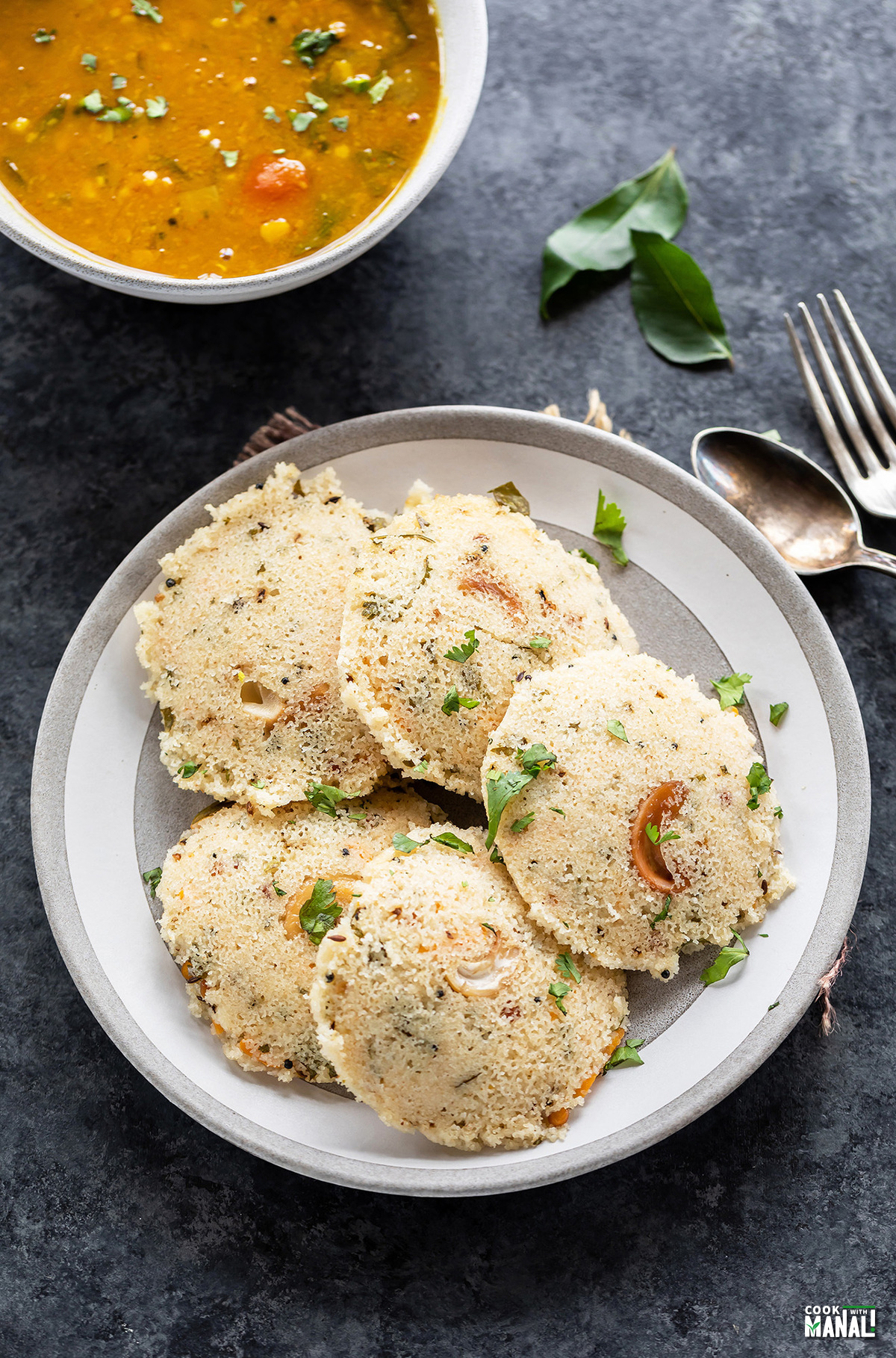The image showcases a plate of intricate Indian food featuring round, UFO-shaped items that resemble a lacy, airy breading with numerous holes, giving it a bloated pancake appearance. The breading, possibly containing nuts like cashews, is garnished with greens and perhaps dried onions or cilantro. These items rest on a striking white and gray plate with a target design. To the right, a fork and spoon are visible, while at the top, a bowl of turmeric-colored dal, adorned with greens, tomato, and possibly corn, adds to the vibrant presentation. The text "Cook Manali" is subtly printed in white at the bottom of the image.